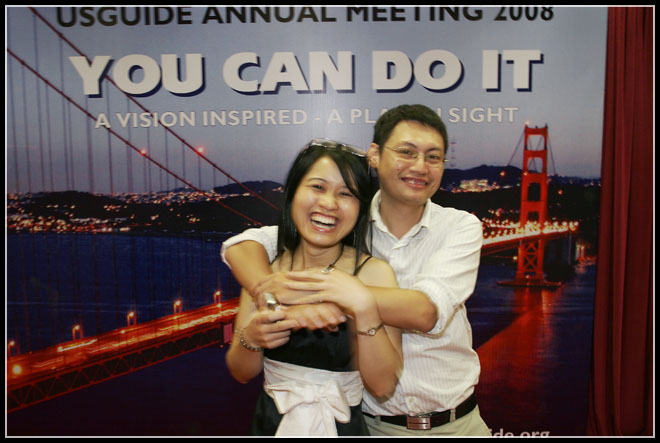A nighttime photograph depicts a young Asian couple in their 20s standing in front of an advertisement. The man, wearing glasses, a white button-down shirt with the sleeves rolled up, and khaki pants, has his arms around the woman. She is smiling brightly and has shoulder-length black hair with glasses perched on her head. She is dressed in a black top with a distinctive white bow around her waist. They are positioned in front of a backdrop featuring a lit-up Golden Gate Bridge, suggesting the image was taken at dusk. The sky is a mix of gray clouds and the fading blue of the evening. The advertisement behind them reads in black and white typography: "US Guide Annual Meeting 2008," followed by the motivational phrases "You Can Do It,” and “A Vision Inspired.” Part of the text, "A-P-L sight," is partially obscured by the man's head. The couple is centered in the frame, smiling at the camera, creating a warm and intimate moment captured against the iconic San Francisco skyline.